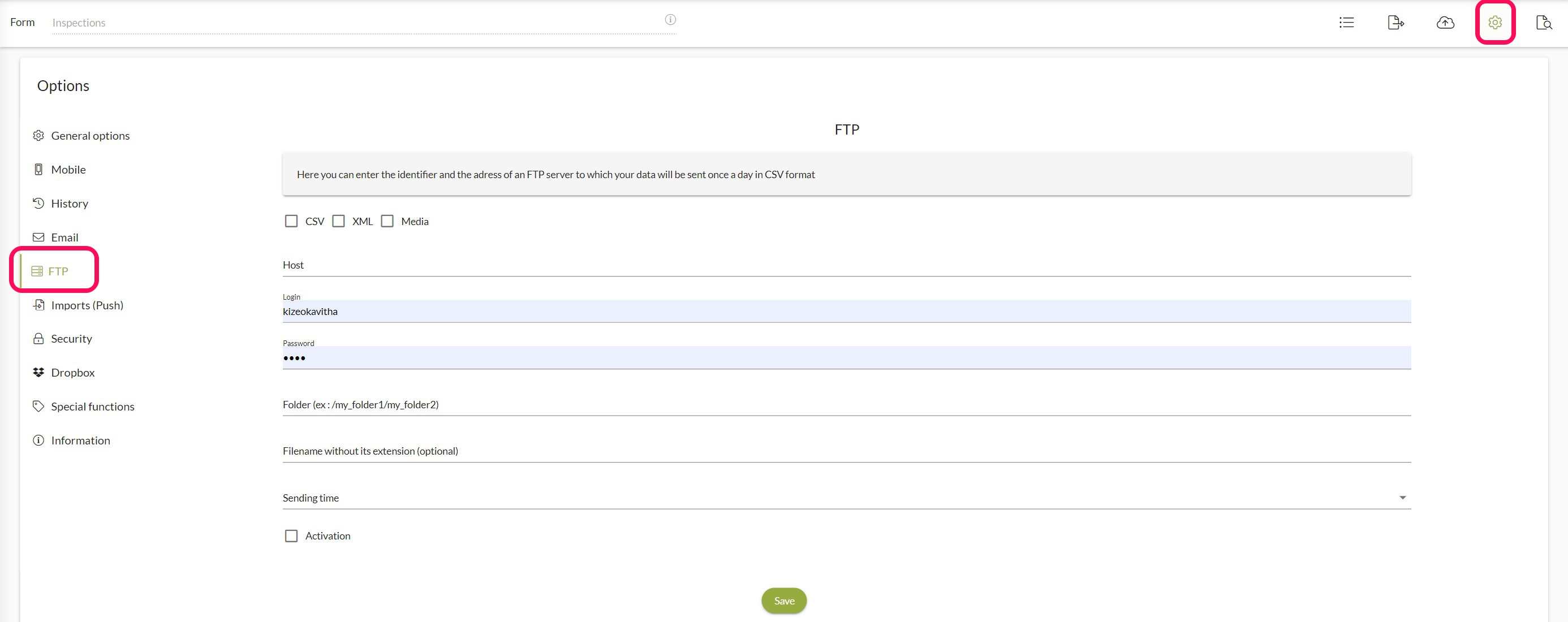The image depicts a recently opened program with a complex and somewhat cluttered interface. The window appears to have been shrunk, causing much of the text and elements to become blurry and difficult to read. 

At the very top, there is a white bar with indecipherable text in the left-hand corner. Below the white bar, a light gray font is visible in a box, though the content is not legible. Adjacent to this box, there is a circle containing additional, unreadable small text.

On the far right side of the interface, there are several navigation options represented by icons rather than text. These icons include:

1. Three horizontal lines stacked on top of each other.
2. A piece of paper with an arrow pointing out to the right.
3. A cloud with an indeterminate element inside.
4. A gear icon, highlighted with a digitally drawn red box, possibly to indicate that it should be selected.
5. Another piece of paper with an unspecified small element inside it.

Below these icons is a large rectangular or square area dominating most of the screen. On the left-hand side of this area, there are several options listed, each accompanied by an icon and a corresponding text label. Within the main body of the interface, various functional options are displayed. The term "FTP" is discernible in this section, indicating fields where a user can enter their login and password credentials.